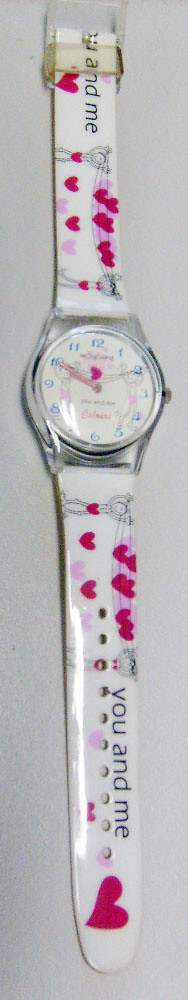This image depicts a white-banded watch with a whimsical and playful design. The band, possibly made of plastic or leather, is adorned with pink and purple hearts and features stick figure characters with hearts concealing body parts, symbolizing beach attire. The phrase "You and Me" is printed on the band in black text. The watch face is white, encased in a silver-toned housing with a clear plastic buckle. The clock face displays blue numbers and features pink hour and minute hands, with a pink heart at the center. A small yellow knob is present on the right side for adjusting the time. The background of the photograph is an off-gray color, and the watch is positioned vertically with the clasp at the top.